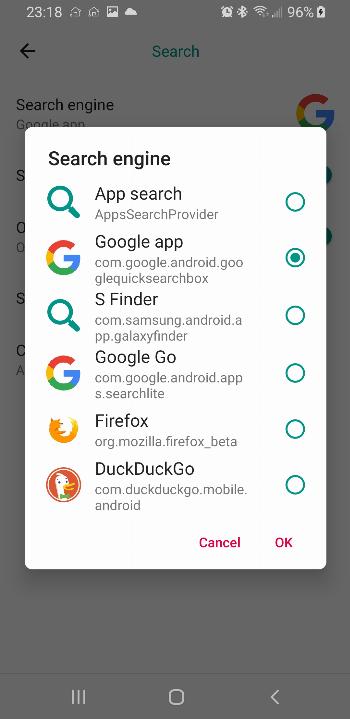A screenshot captures a pop-up window on a user's darkened cell phone home screen, emphasizing the pop-up in a prominent white vertical rectangular box. The top section of the home screen reveals system details: the time displayed as 23:18 on the left, with various icons indicating the user's phone status on the right. Among these, there's a battery level at 96%, an active alarm, and a single signal bar.

The pop-up is titled "Search Engine" in bold black text. Within the pop-up, a vertical list of selectable options is presented. Each option includes an associated icon on the left and a selection button on the right. The listed options are: 
1. **App Search**
2. **Google App** - with a filled green selection button indicating it is currently selected.
3. **S-Finder**
4. **Google Go**
5. **Firefox**
6. **DuckDuckGo**

Each option also features a brief light gray description beneath it. At the very bottom of the pop-up, there are two actionable text options, "Cancel" and "Okay," displayed in purple.